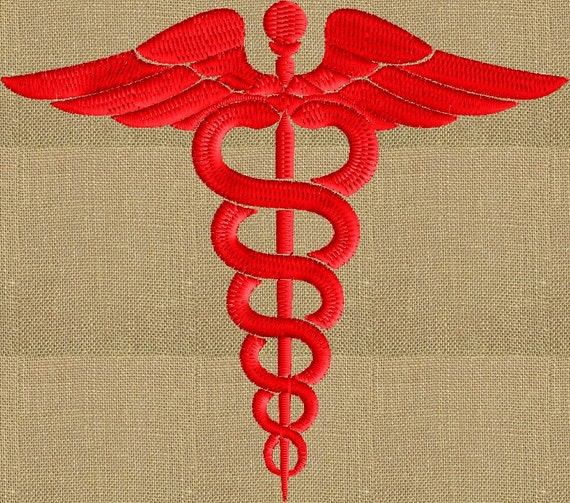The image features a detailed and meticulously stitched symbol prominently displayed against a textured beige cloth background. This cloth appears to be canvas-like and exhibits gradations of brown, transitioning from a darker shade at the top to a lighter beige at the bottom. The focal point, occupying the central space of the picture, is a red symbol that bears a strong resemblance to the caduceus, a common emblem in the medical community. This symbol consists of a vertical staff topped with a spherical element and flanked by wings at its apex. Two serpents coil intricately around the length of the staff, their heads meeting near the top, just below the wings. The cloth and symbol exhibit fine craftsmanship, with visible small stitching in both the beige fabric and the red thread of the symbol, suggesting it is handmade and possibly conveys an important affiliation or thematic representation.